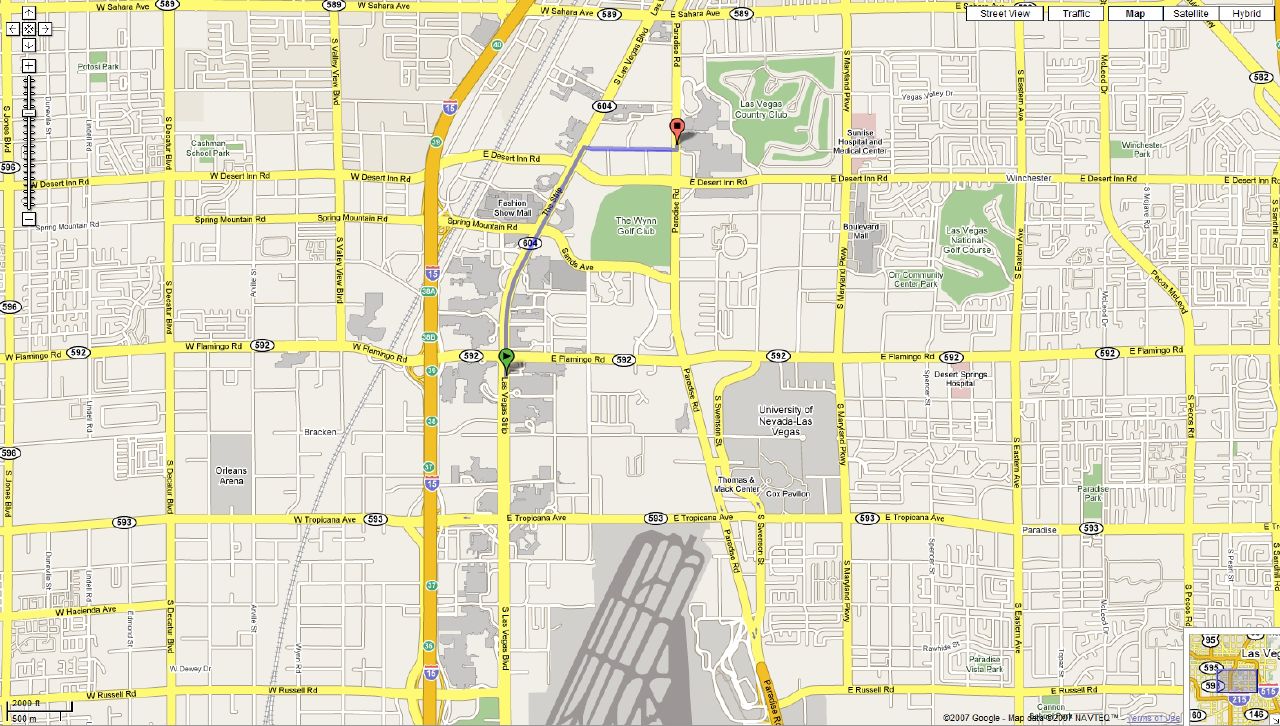This detailed city map of Las Vegas provides a close-up view of a specific section of the city, prominently featuring the University of Nevada, Las Vegas campus. The map highlights several noteworthy locations, including the Wynn Golf Club with its lush green fairways. Major city streets and intersections are clearly marked, illustrating the intricate layout of the urban area. Various parks and points of interest are also identified, adding to the navigational utility of the map. The streets are color-coded with main streets in yellow and side streets in white, typical of a MapQuest-style presentation.

Additionally, a specific route is plotted on the map, starting from a location along Las Vegas Boulevard and heading towards the Las Vegas Country Club, suggesting a point of interest or destination for travelers. A highway is visible, snaking through the area and connecting different parts of the city. Overall, this map serves as a comprehensive guide for navigating this bustling section of Las Vegas.